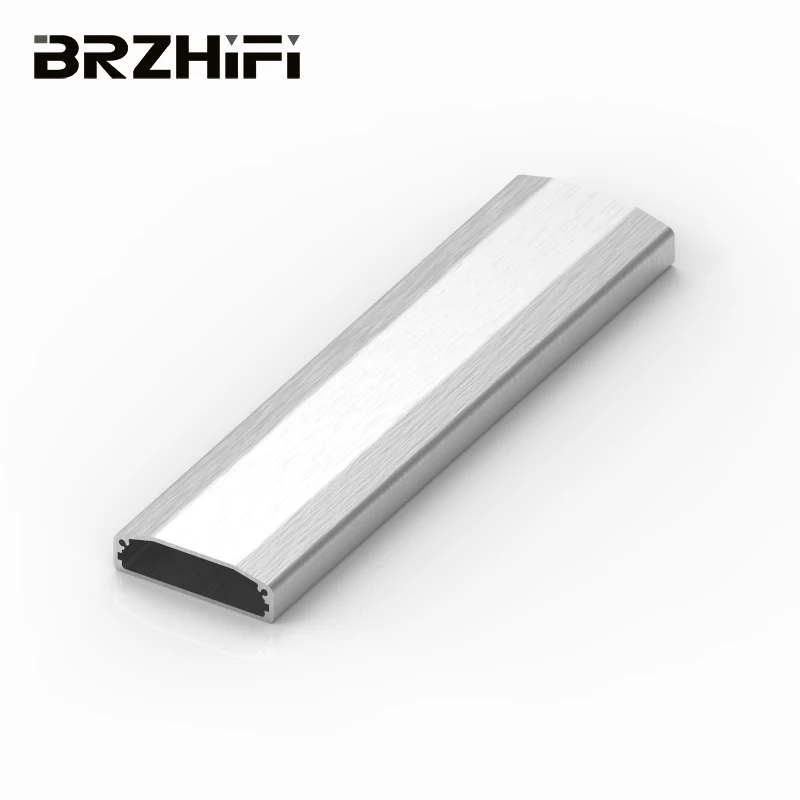The image features a small electronic component that resembles a memory stick, prominently displayed on a white background. The component has a distinctive silver and gray metallic appearance, with a textured surface that almost resembles wood. One end of the component is solid black, possibly hollow or filled in. At the other end, there is a noticeable white strip where light is reflecting off the surface. The upper left corner of the component is marked with the logo "B-R-Z-H-I-F-I," written in stylized, all-capital letters with unique design elements; notably, the I's are dotted with upside-down triangles and the B and F have intricate graphic features. This piece is shaped somewhat like a flat rectangle with a flattened cylindrical form and is approximately five to six inches in length. It appears to serve a functional purpose, possibly as a connecting clip for different parts, and might be found in contexts such as automotive dashboards.